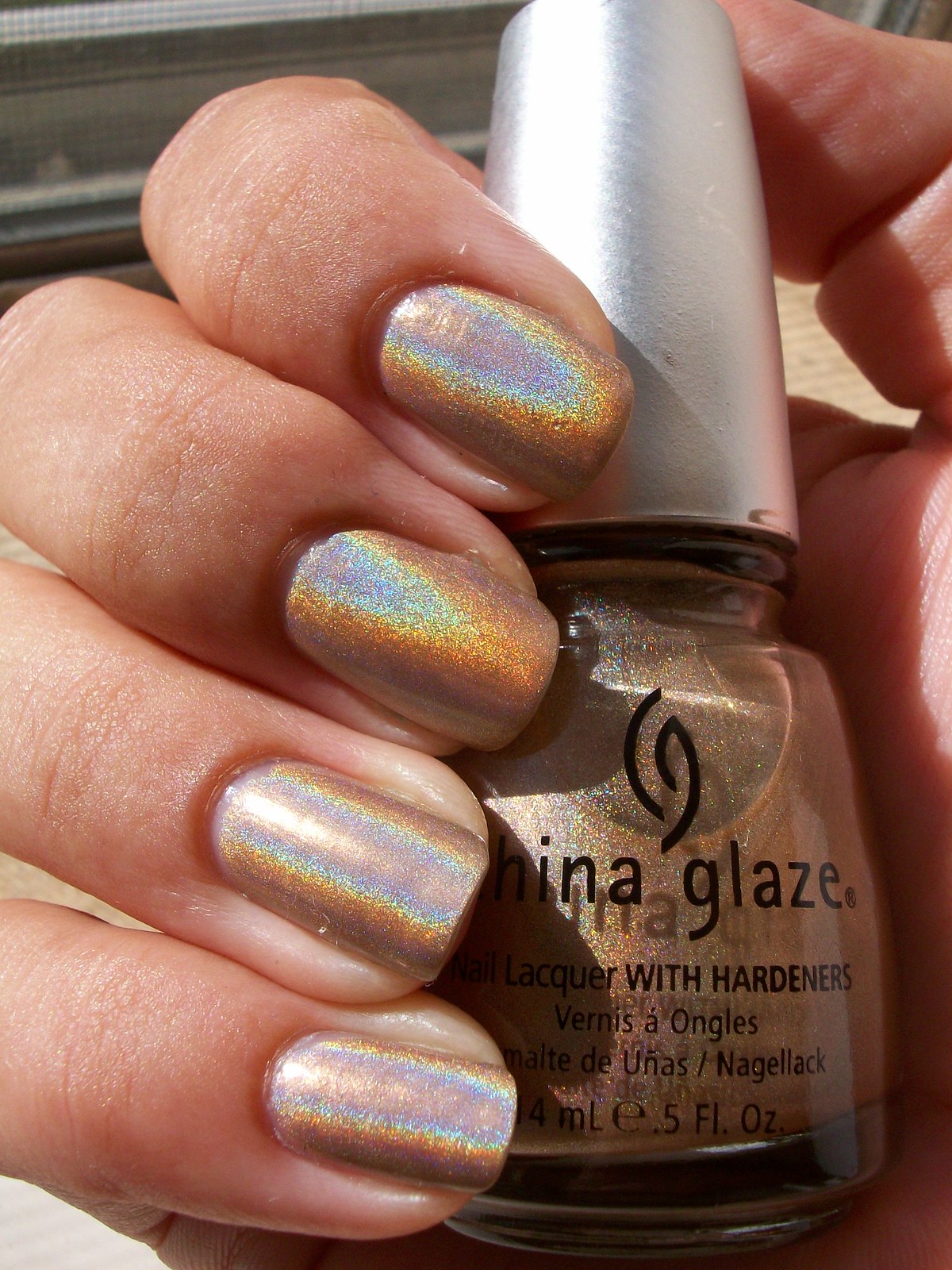This close-up image features the right hand of a Caucasian woman showcasing her stunning holographic nail polish, which presents a severe, rainbow-like effect. She is holding a bottle of China Glaze nail lacquer. The holographic nail polish on her fingernails and the bottle she's holding both exhibit a metallic, sparkly gold shade. The glass bottle features black text and branding, with a silver, swirl-logo-embossed twist-off cap. The label on the bottle reads "China Glaze," followed by "Lacquer with Hardeners" and "Vernis à Ongles" in another language. The bottom line of the label displays "4 mL / 0.5 FL OZ."